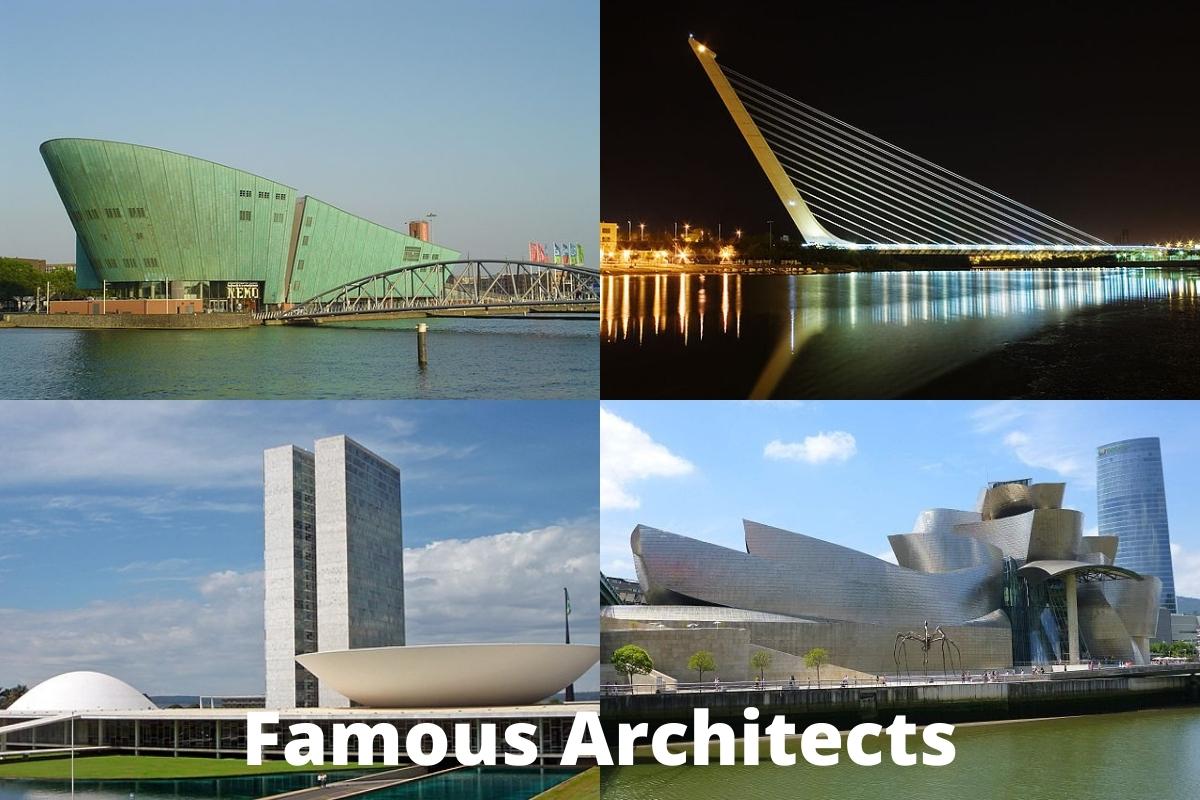This rectangular image is divided into four quadrants, each showcasing a different photo of iconic architectural structures under the collective title "Famous Architects" displayed in white text at the bottom. The top left quadrant features a green-tinted, dome-shaped building adjacent to a bridge, set against a body of water. The top right quadrant displays a structure with white lines likely forming part of a triangular bridge that stands over water, highlighted dramatically against a dark background with reflections suggesting a night view. The bottom left quadrant presents two tall, thin rectangular towers flanked by a white dome on the left and a white bowl-shaped structure on the right, all beneath a clear blue sky. The bottom right quadrant reveals a silver, curvilinear building with a blue sky and green water, accentuated by an artistic sculpture, potentially resembling a giant spider, in front of it. The vivid colors—blue, green, brown, yellow, grey, white, and black—enhance the visual appeal of these well-positioned photographs, making it an ideal display for architecture enthusiasts.